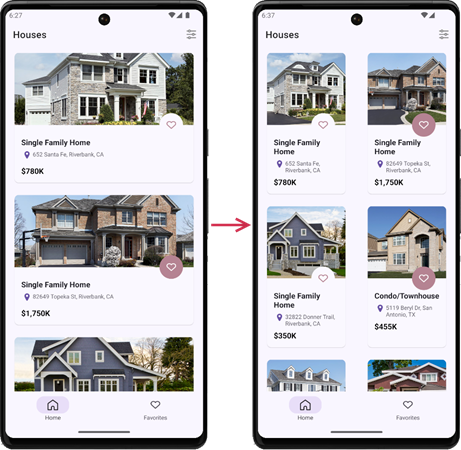The image depicts two smartphones positioned side-by-side, both showcasing black borders and white screens. An arrow, colored in a vivid purple hue, stretches between the two devices, indicating a transition from the left to the right. At the top center of each screen, a black circle is prominently displayed.

On the left smartphone, the screen displays a section titled "Houses." Below this title, there is a detailed image of a two-story gray house with an attic window, surrounded by trees. The house is labeled as a "Single-Family Home" with an address located in California, and is priced at $780,000. Further down, another listing showcases a brick house with a basketball hoop positioned in front of the garage. This property is also marked as a "Single-Family Home" but comes with a significantly higher price tag of $1.75 million. 

On the right smartphone, the screen mirrors the layout but features a quaint, small purple house with a white border encircling the roof, providing a sense of charm and uniqueness to the property display. The setting and context imply a comparative or transitional scenario between the two devices, potentially involving real estate browsing or an app function.